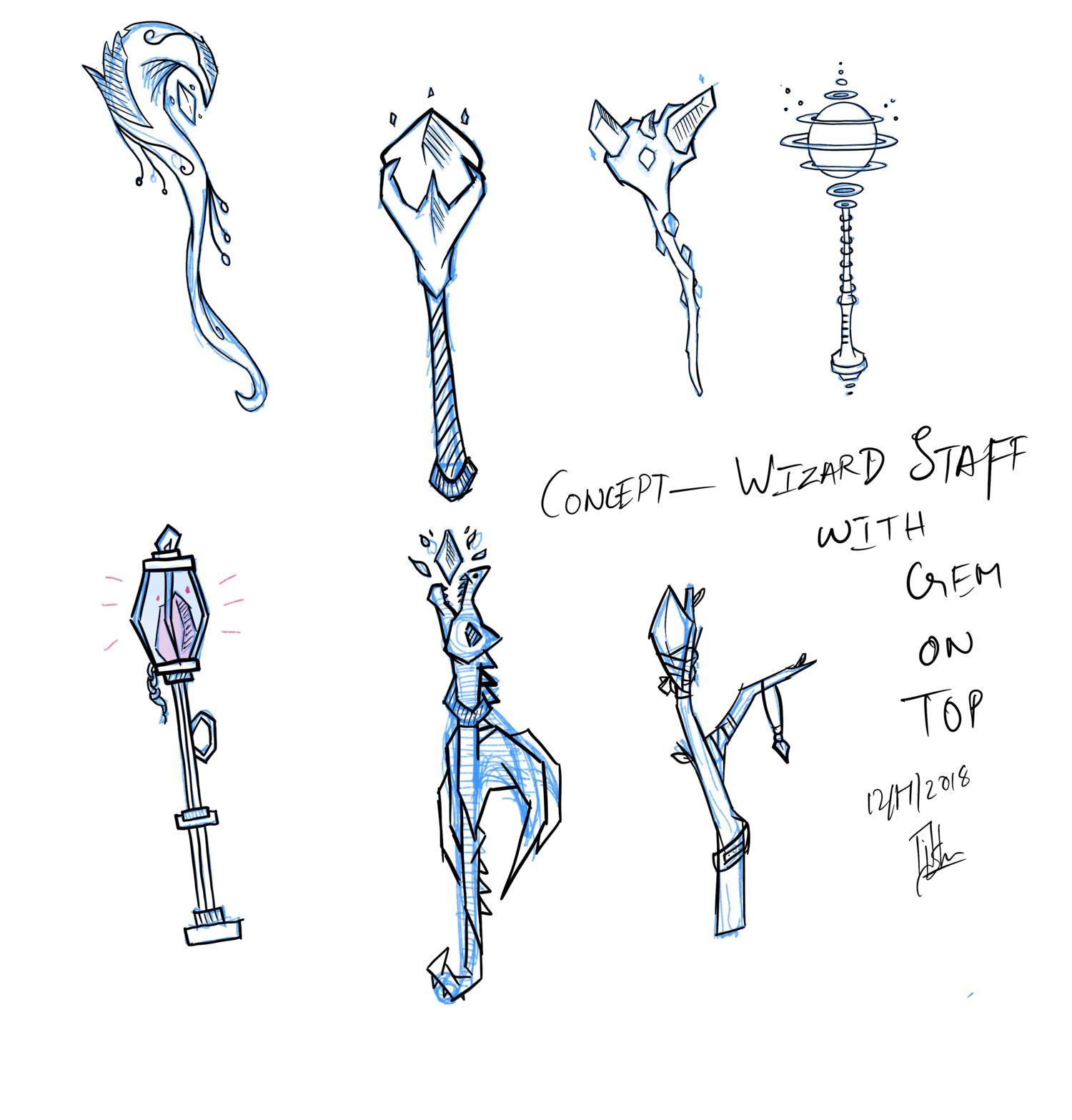This hand-drawn concept art, dated December 17, 2018, showcases seven variations of wizard staffs, with "Concept Wizard Staff with Gem on Top" handwritten in the lower right-hand side beside a signature. The artwork is divided into two rows: four staffs on the top and three on the bottom, all set against a white background. Each staff features unique and intricate designs reflecting an array of magical aesthetics. The top row includes a staff that appears to have a curvy, wood-like structure, a straight staff holding a stone within a four-pronged holder, a double-horned staff, and one resembling the planet Saturn, detailed with three rings around a ribbed pedestal. The bottom row continues with creative designs, including a staff that looks like a street lamp with a crystal inside a lantern, a serpent-long with a gem, and a figure that suggests a woman dancing, kicking her legs. These silhouettes, tinted in a faint blue hue, encapsulate a whimsical and fantastical vision of wizardry.